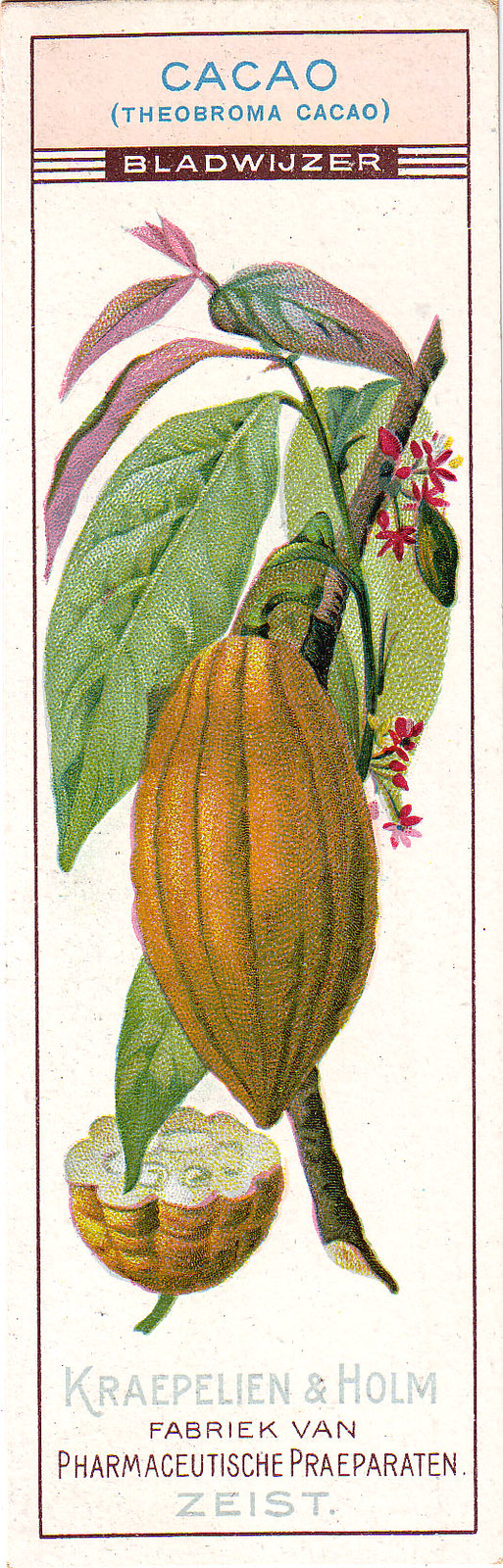This image is a tall, narrow vintage illustration containing botanical details and descriptive text. It features a vibrant color depiction of a cacao pod on a brown stem with green leaves and small red flowers. The cacao pod is a vivid brown hue, partially cut open to reveal a white, fluffy, fleshy interior with slight green tints. The illustration shows the pod in close-up, highlighting its intricate textures and structures.

At the top of the image, there is a pink horizontal band with blue text that reads "Cacao" followed by "(Theobroma cacao)" in parentheses. Just below this, a narrow dark brown stripe contains white text that states "Bladwijzer." The main illustration occupies the cream-colored background, vividly displaying the botanical characteristics of the cacao plant. Toward the bottom, further text reads "Kraepelin and Home" followed by "Chemische Präparaten," indicating that the image likely originates from a non-English source. The overall style combines graphic design with watercolor wash or pastel crayon techniques, creating an aesthetically pleasing botanical illustration.